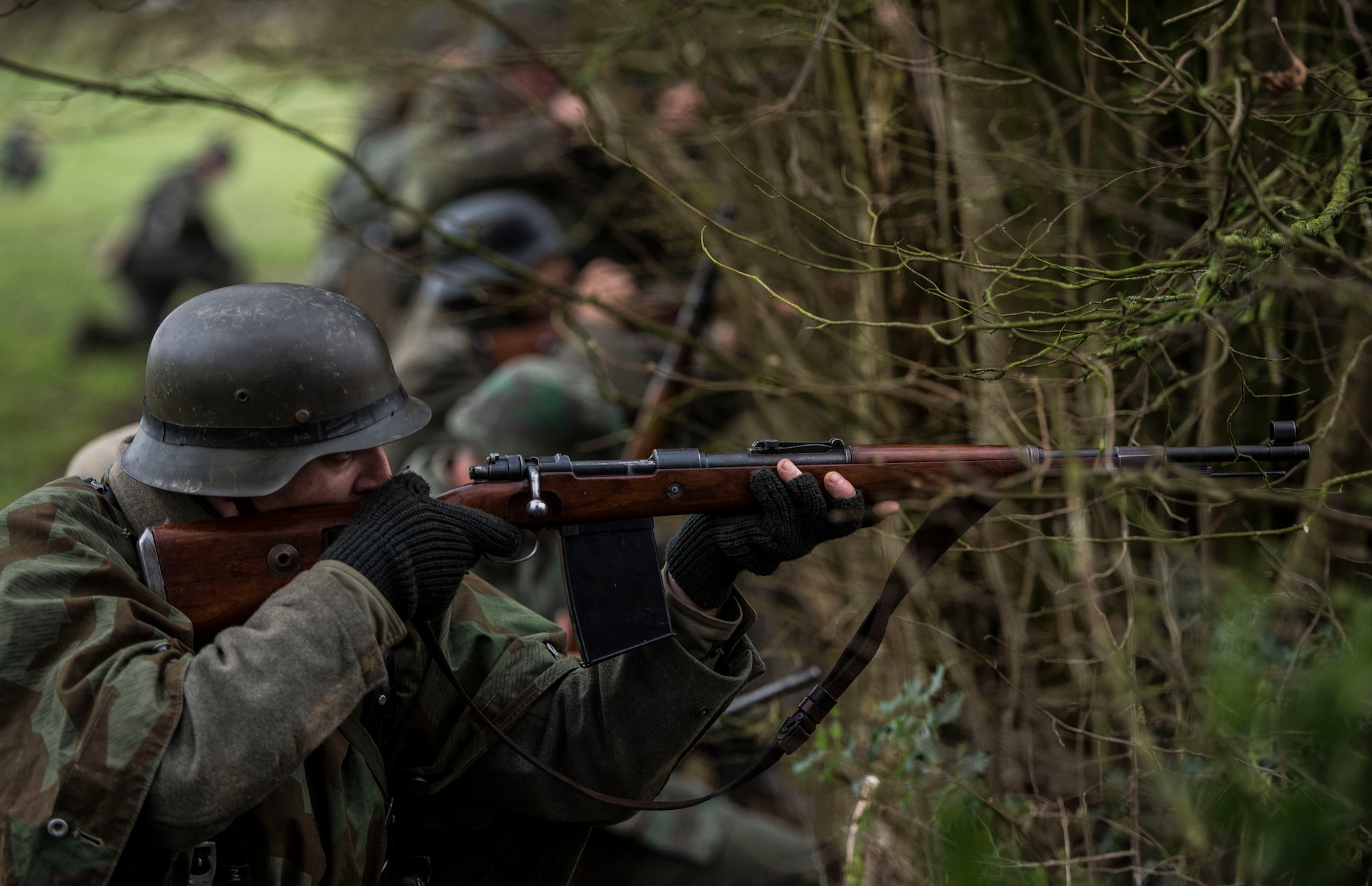The image features a group of soldiers, primarily centered around one prominently focused soldier in the lower left of the frame. This soldier is equipped with a gray helmet and an army fatigue jacket over a gray shirt, and is wearing black gloves with cut-out fingers, revealing his fingers. He holds a rifle with a wooden stock and black components, including a black strap that drapes from the middle of the rifle underneath his right hand. His right hand is on the butt of the rifle with his finger on the trigger, aiming purposefully straight ahead. His left hand supports the rifle beneath the stock.

In the background, a line of soldiers stretches up towards the top left corner of the image, though they appear blurry and indistinct. These additional soldiers are clad in various green, brown, and black camouflage uniforms, and some are kneeling amidst a grassy terrain interspersed with patches of bare mud. Most of the background is obscured by tree branches, sticks, and stems, creating a dense thicket on the right side of the image. Additionally, there is noticeable greenery including bushes in the bottom right corner and sparse green leaves among the bare branches.

Despite the blur, it is clear that all soldiers are intently focused on aiming their rifles towards the dense tree line ahead, possibly engaging an unseen enemy. The entire scene is framed by the natural, somewhat chaotic mess of the woodland area, enhancing the tension and urgency of the moment captured.